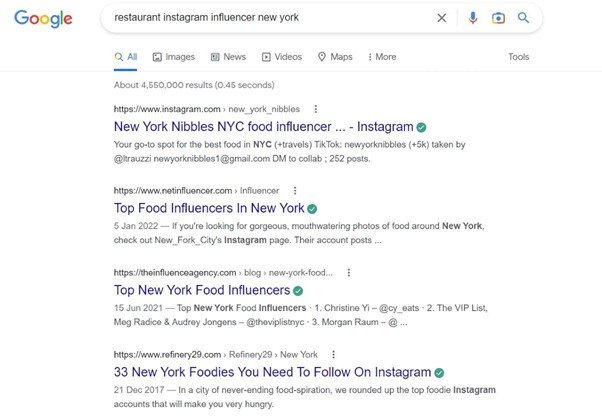A detailed screenshot of a Google search results page for "Restaurant Instagram Influencer New York." The search term is displayed prominently in the search bar at the top. Just below the search bar, the conventional navigation tabs for "All", "Images", "News", "Videos", "Maps", and "More" are visible, with "Tools" located to the right of these options.

The first search result is titled "New York Nibbles NYC Food Influencer Instagram" followed by a short description in a lighter gray font. The second result is titled "Top Food Influencers in New York," also accompanied by a brief description. The third result, "Top New York Food Influencers," includes a similar description style. Each of these results is marked with a green circle and a checkmark icon next to the title, indicating their authenticity or verification.

The fourth search result stands out with the title "33 New York Foodies You Need to Follow on Instagram." Its description reads, "In a city of never-ending foodspiration, we rounded up the top foodie Instagram accounts that will make you very hungry." This description emphasizes the allure and appeal of these curated Instagram accounts for food enthusiasts.

Overall, the screenshot gives a comprehensive overview of the top search results for Instagram food influencers in New York, providing a clear guide for anyone looking to explore popular foodie accounts in the city.